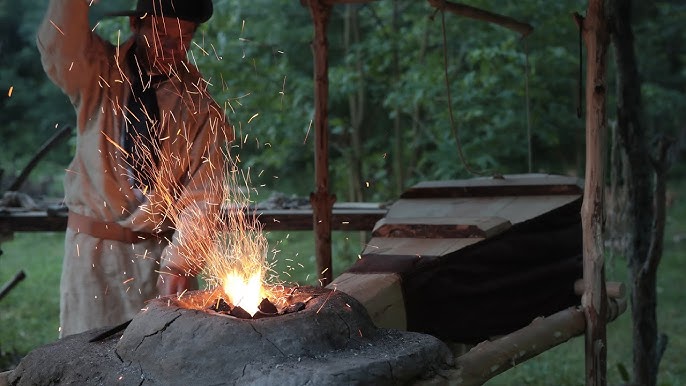In this detailed, landscape-oriented color photograph, we see an outdoor scene featuring a blacksmith at work within a rustic, open-air shelter made of tree logs. The shelter, designed to avoid catching fire, houses a variety of wooden structures, including a large rectangular bellows prominently positioned on the right side of the image. The focus is on the blacksmith, an Asian gentleman dressed in a green robe, standing on the left side of the photo. He is visible from his mid-head to his mid-hip and appears poised to strike an unseen instrument with his arm raised above his head. 

At the center of the scene, before him, lies a round, low, concave structure reminiscent of a well, filled with hot coals. Bright yellow flames and fiery sparks erupt from this structure, illuminating the area and casting a dynamic display of light. The surrounding ground is covered in green grass, and the image is framed by a backdrop of dense, verdant trees, emphasizing the natural, forested setting. This highly detailed photograph beautifully captures the essence and intensity of the blacksmith's craft amidst a lush woodland environment.